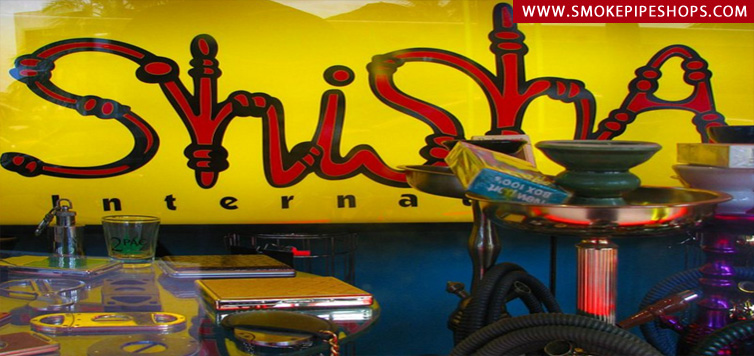The image depicts a vibrant scene inside a hookah bar, marked by a bright yellow background wall adorned with red lettering. The top part of the text spells out "SHISHA" in a script resembling a hookah hose, while below it reads "INTERNA" in black letters, though it's partially obscured. Dominating the foreground on the left side is a shiny glass table, upon which lies a tan book and another partially visible book. Also on the table is a short drinking glass emblazoned with "Tupac". The right side showcases two hookahs: the foremost hookah has a vibrant purple stem and a green pot at its top, while the second one presents a dull silver finish with a black hose and a yellow and blue box marked "Box 100". The base of the image reveals a bluish floor that contrasts with the vibrant yellows and reds above, hinting at the lively atmosphere of the hookah bar.